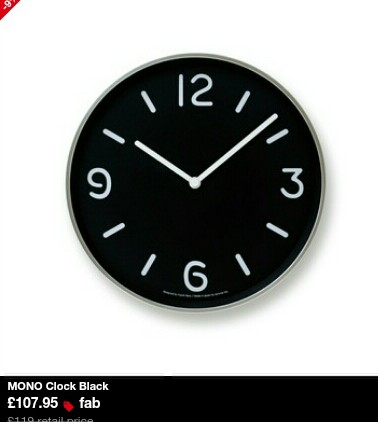This image appears to be an advertisement for a minimalist wall-mounted clock. The background is completely white, providing a clean canvas to highlight the clock and associated details. The clock itself is round with a simple gray bezel and a black face. Prominently displayed are the numbers 12, 3, 6, and 9 in white, while the remaining hours are marked with white dashes. The clock shows the time as approximately eight minutes past ten. Both the hour and minute hands are simple white rectangles.

In the upper left corner of the image, there's a small red triangle that partially displays a "G". The lower portion of the image features a black rectangular bar spanning from left to right, containing the text "Mono Clock Black" in white letters, along with the price £107.95. Nearby, there's a small red icon with the word "FAB" in white, adding a touch of color to the minimalistic design. Other than these elements, there are no additional words, text, or graphics visible in the image.